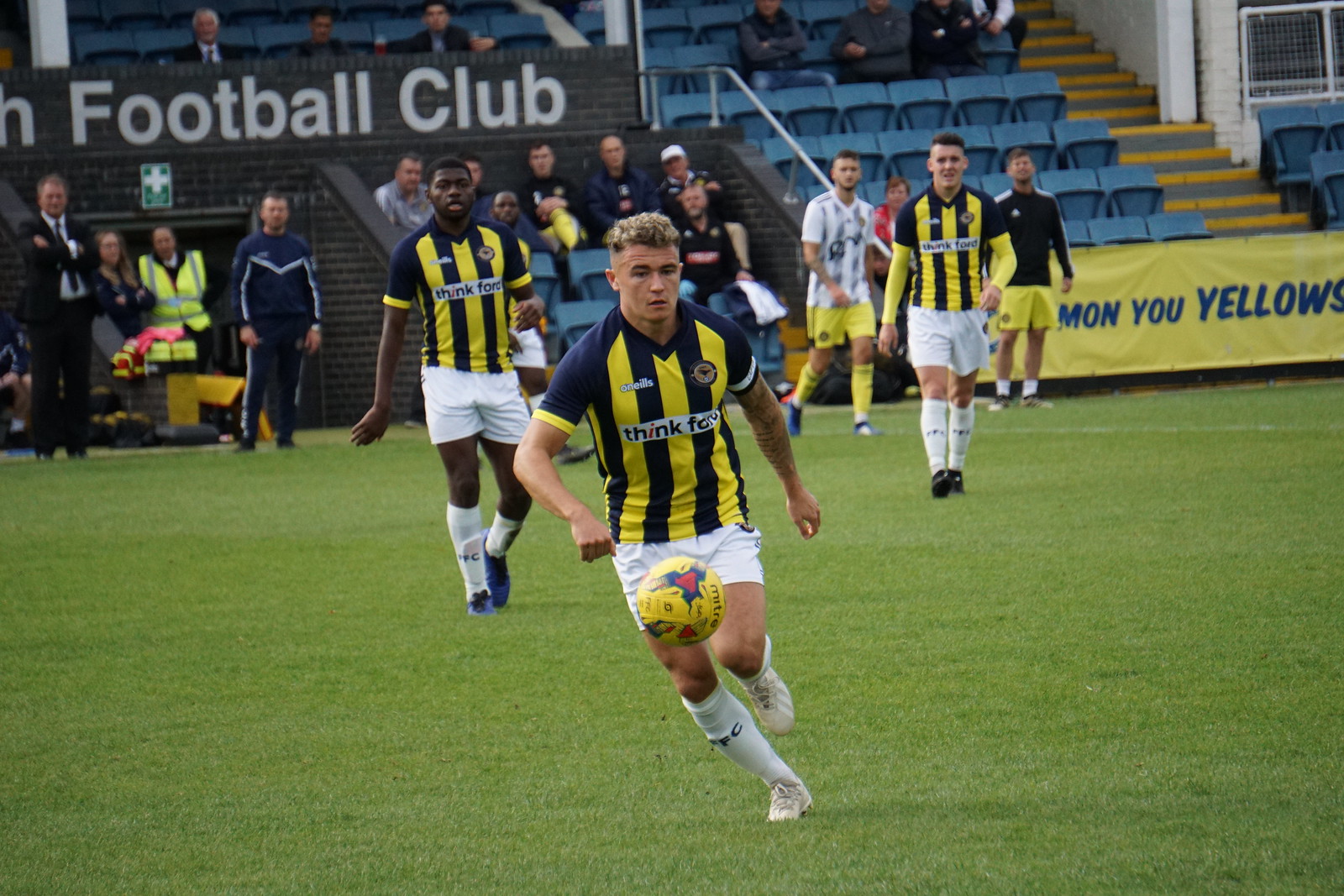In this detailed image, a group of men is playing soccer on a vibrant green field. The central figure is a player with short, blonde, curly hair on top and shaved sides, intently focused on a midair yellow soccer ball around crotch level. He wears a navy blue and yellow striped uniform with the sponsor "Think Ford" visible on the front, paired with white shorts and white socks. Surrounding him are three other players in similar black and yellow vertically striped shirts and white shorts. An additional player further back sports a white shirt and yellow shorts. In the background, blue-seated stands are partially occupied, with most spectators and additional figures gathered off to the side of the field. Notable visible text includes a partially obscured "In Football Club" and "Monu Yellows" on a right-hand banner.